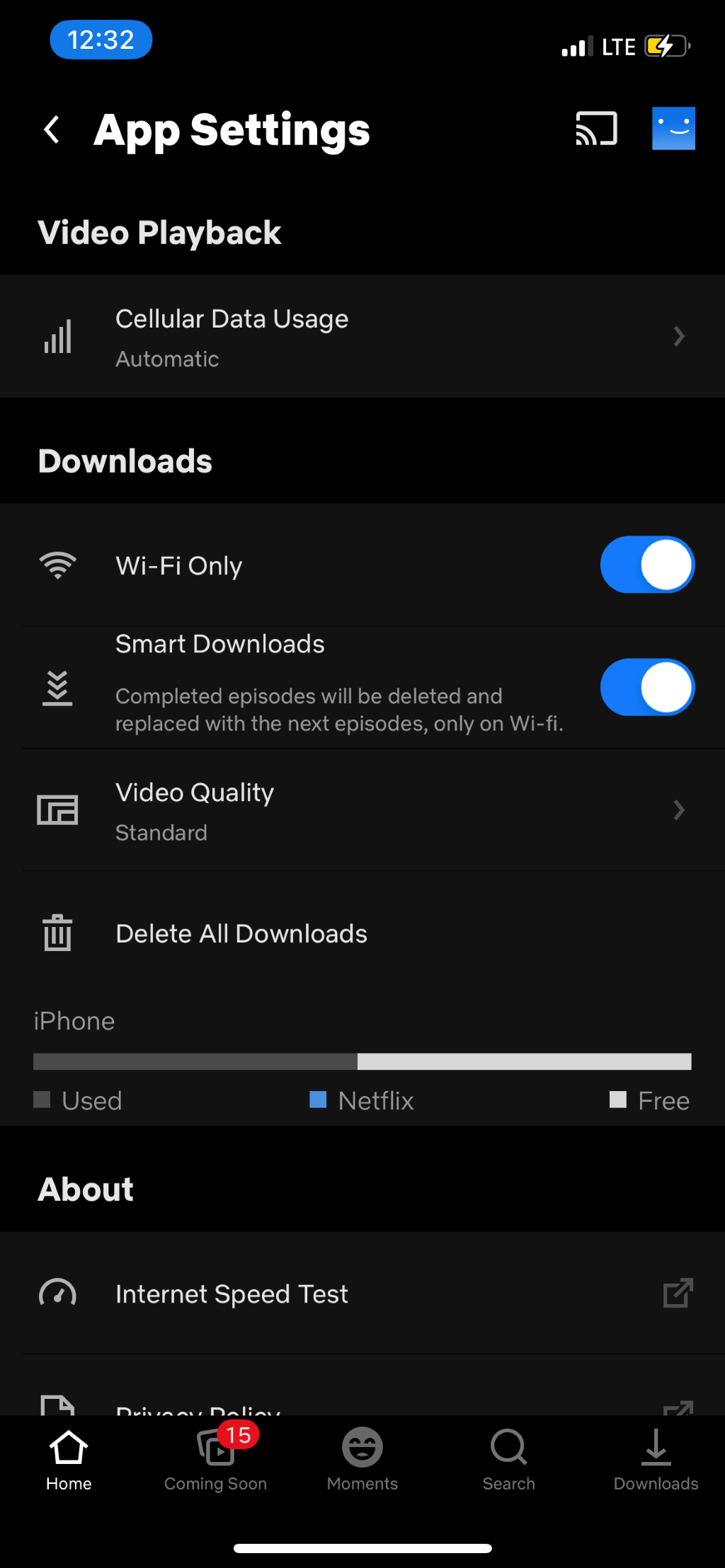**Detailed Caption:**

This is a vertical portrait screenshot of a smartphone displaying an app settings page. At the top of the phone's screen, the status bar shows the time as 12:32, an almost full LTE service bar, and a charging battery icon that is about halfway full. The title of the page reads "App Settings." To the left of the title, there is a back button; to the right, there are icons for screencast and account settings.

Underneath the title, the first section is labeled "Video Playback." Here, the cellular data usage is set to automatic. Below this, in the "Download" section, the "WiFi Only" option is turned on, and the "Smart Downloads" option is also enabled. The latter is described as a feature where completed episodes will be deleted and replaced with the next episode only when connected to WiFi. Following these settings, the "Video Quality" option is set to standard.

Further down, there is a "Delete All Downloads" button. Proceeding below this, a storage meter for the iPhone indicates that the used space is about halfway full. At the bottom of the screenshot is an "About" section, which includes buttons for tasks such as conducting an internet speed test and several navigation icons.